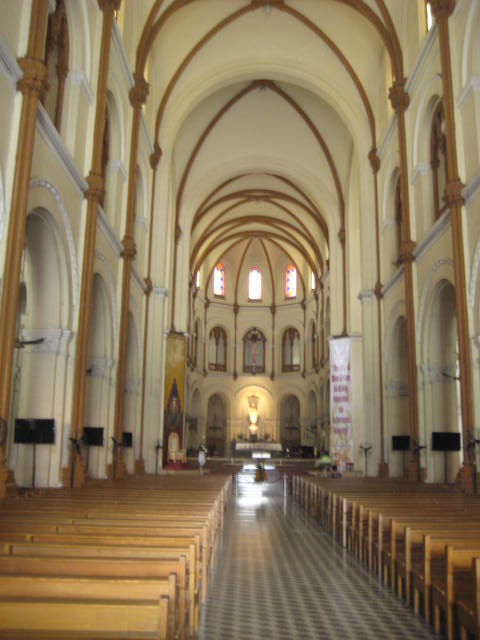This photograph, taken from the back of a narrow church or basilica, captures the central aisle between beige wooden pews leading up to the altar. Dominated by a white palette with subtle beige trim, the space features unique architectural elements including high, arched ceilings adorned with brown curved lines and vertical posts descending down the walls. Despite the minimal religious iconography, stained glass windows high up filter light into the space, making their designs somewhat indistinguishable. The black and white checkered floor of the central aisle draws the eye towards the well-lit altar, which, though devoid of traditional religious symbols or images of Jesus, holds an understated yet powerful presence at the end of the aisle.